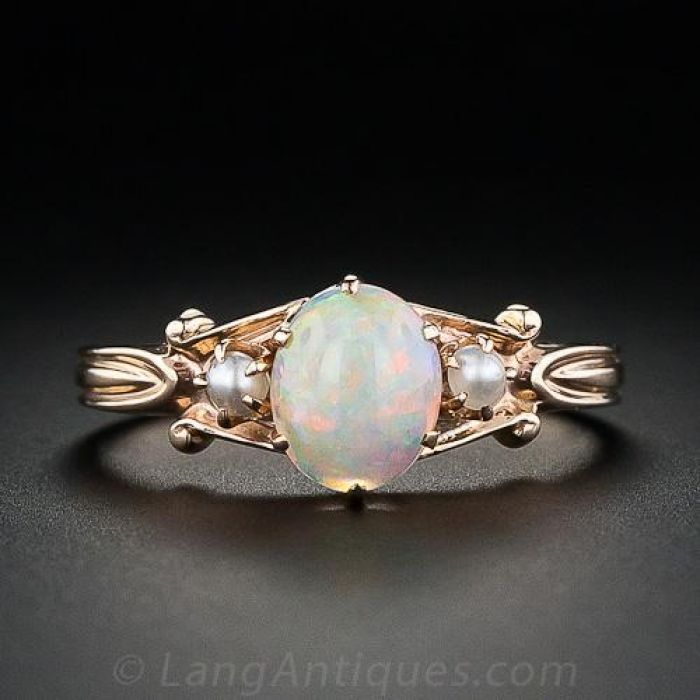This interior photographic image captures a stunning antique gold ring, prominently displayed against a grey background with a watermark reading LangAntiques.com at the bottom. The centerpiece of the ring is an opal stone, oval in shape and exhibiting a mesmerizing iridescence with shades of green, blue, pink, and purple. Flanking the opal on either side are two half-dome pearls, each securely held by four delicate golden clasps. The ring's band is elegantly tapered, widening outward to support the opal, which is firmly held by five clasps. The background is grey, adding a subdued contrast that highlights the intricate details and craftsmanship of the ring.